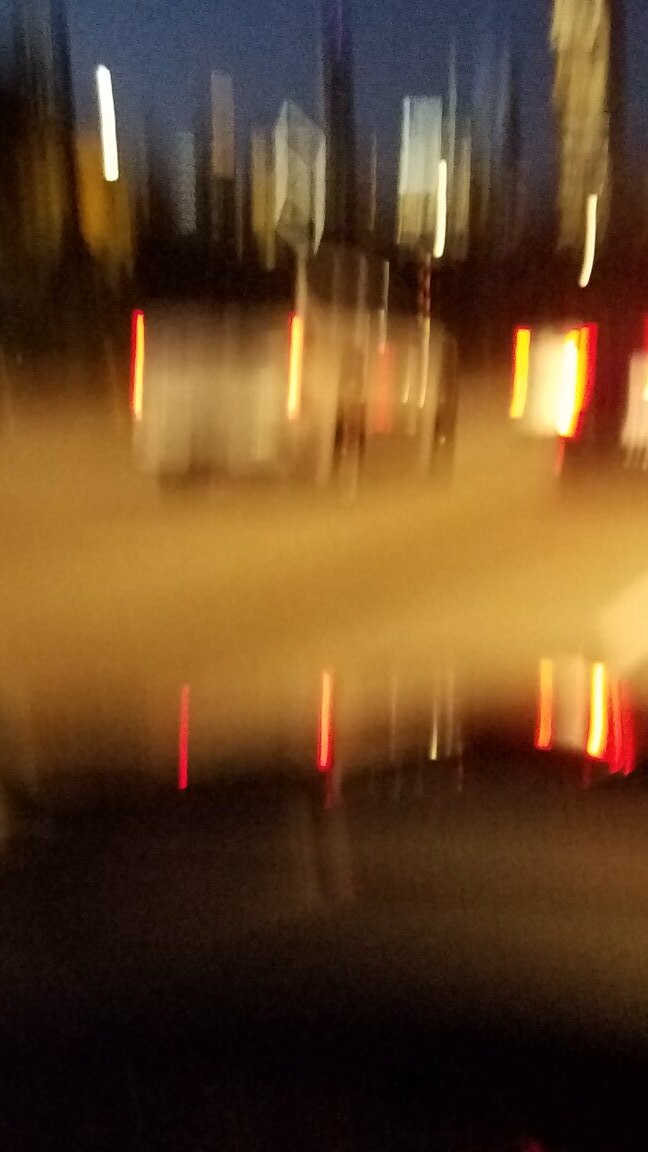The image is a blurry photograph captured from inside a car, possibly using a dash cam. The bottom part of the image is black, resembling a car dashboard with potential reflections or lights. The main focal point is a white vehicle, likely a truck or SUV, approximately 30 feet ahead. This vehicle's red brake or running lights appear as distorted vertical lines. The scene extends to a vague city skyline with indistinct skyscrapers and possibly a lamppost to the right. Additionally, there seems to be another car in front of the white vehicle, possibly a smaller model like a Prius. Overall, the image is marked by significant blurriness, affecting all elements, including the roadway and surrounding structures.